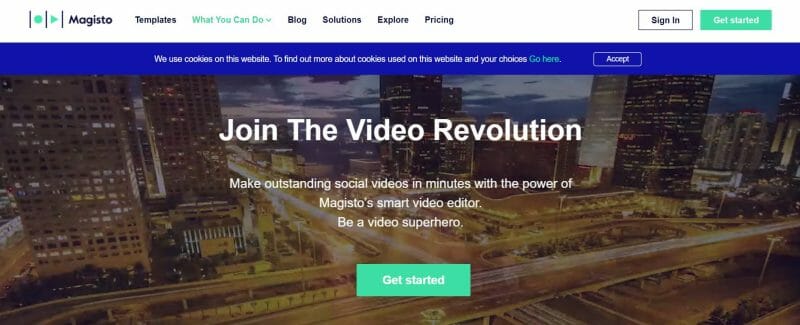The video showcases the homepage of Magisto, a popular video editing platform. At the top of the screen, there is a blue strip containing various navigational options such as "Templates," "Blog," "Solutions," "Explore the Website," "Pricing," "Sign In," and a prominent green "Get Started" button. Below this navigational bar, the screen features a vibrant image of a bustling city with major thoroughfares, overlaid with text that reads: "Join the Revolution. Make outstanding social videos in minutes with the power of Magisto's smart video editor. Be a video superhero. Get started." Additionally, a prompt about cookie usage appears, offering users the option to learn more or accept. The section highlighted in the navigation bar is "What You Can Do," encouraging users to sign in and start creating their own videos.